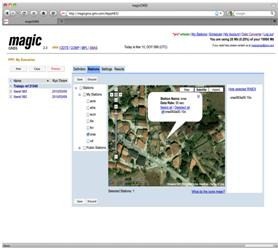This image appears to be a screenshot taken from a computer screen, as indicated by the presence of a solid gray bar at the top with two search bars positioned in the middle. The screenshot seems to display a webpage for a company named "Magic," which may be related to real estate or property tracking. The word "Magic" is written in small case, bold black letters, with some purple text to its right, followed by additional small black letters.

Further to the right, there's a section with multicolored script containing green, blue, and black letters, though the text is too small to decipher. Below this section, there are numerous options, with the main focus being an aerial view of several homes in the center of the screen. A particular home is highlighted, and its details are magnified in a chat bubble-like format.